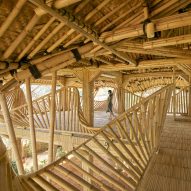The image captures a unique, tan-to-brown wooden deck that is covered by a roof made of wooden beams and circular boards, with a thatched, needle-like roofing material. The deck features a very distinct railing system, with the railings leaning and curving whimsically, almost like a roller coaster. One railing in the foreground curves dramatically to the left and then arches up to the right, while the railings in the background continue this wavy, topsy-turvy pattern, giving an impression of a structure that is almost crumbling or collapsing inward. In the center of the image, a person stands on the deck, out of focus, adding a sense of scale and depth. The deck flooring is a darker brown wood, and green plants can be seen set against the tan floor, enhancing the natural feel of the scene. The background reveals a white setting and indicates that the deck is on the second floor, as another floor is visible below.